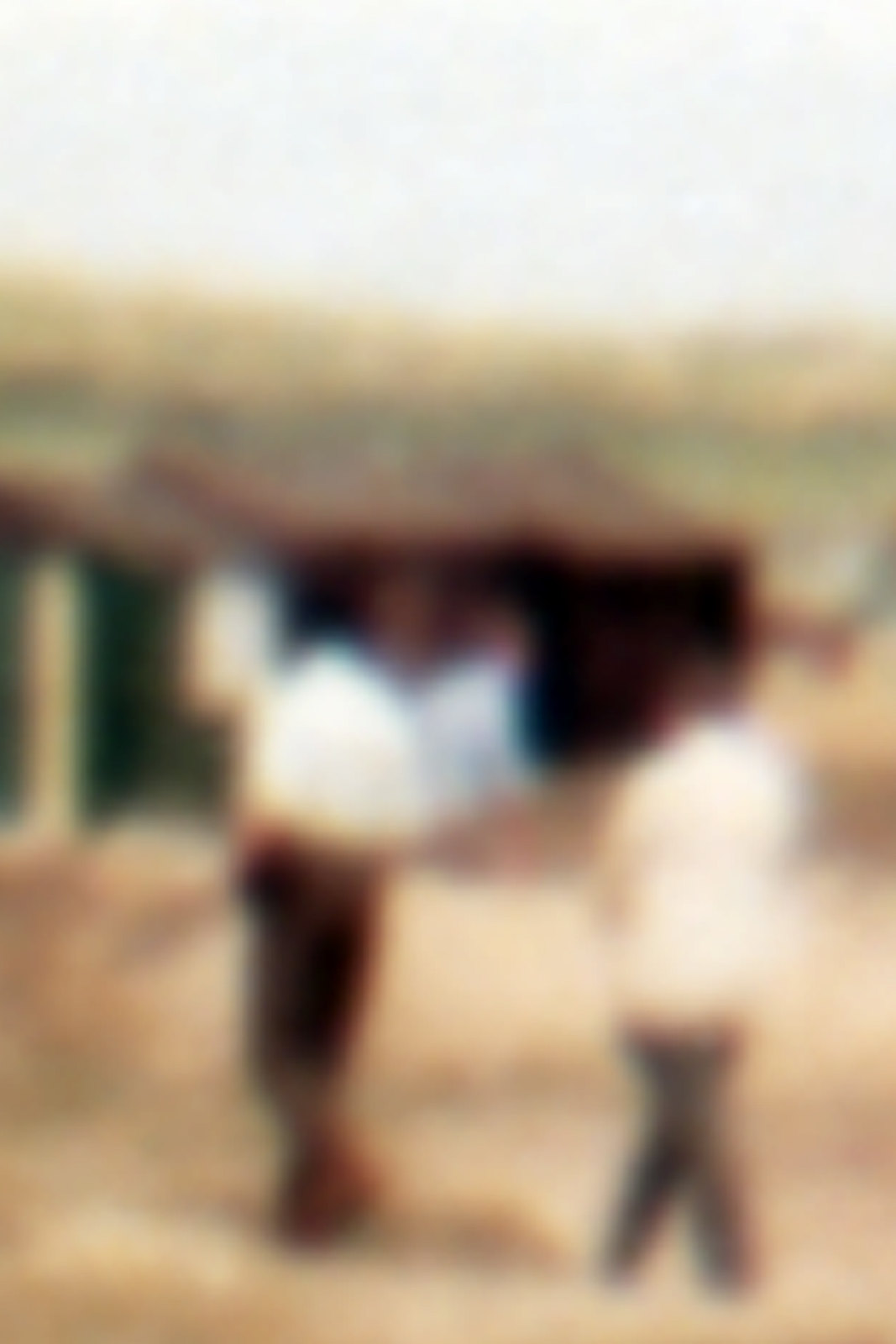Despite the blur, this image clearly portrays two individuals dressed in white tops. The first person is wearing dark brown pants, while the second is in lighter gray pants. They appear to be walking on a dirt path or ground, with distinctive body language suggesting the individual in front may have their hands in their pockets. In the backdrop, there are two contrasting buildings; one is green and white, and the other has a rustic, brown wooden appearance. The scene extends into the distance with a verdant touch, hinting at some green foliage or landscape.